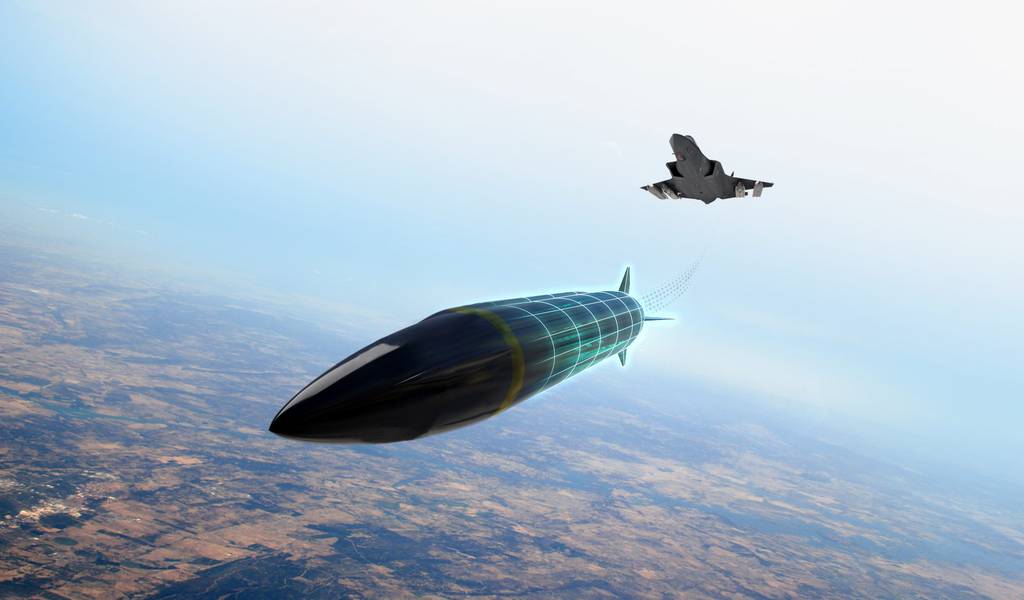This detailed digital render captures a high-altitude scene featuring a grey fighter jet in flight. The jet, seen primarily from below with some white underwing markings, has just fired an intricately depicted missile. The missile's design includes a shiny, black metallic tip, a yellow circular stripe, and a distinctive turquoise and light blue cylindrical body wrapped in a white mesh grid pattern, giving it a high-tech appearance. A stream of dots connects the back of the missile to the jet, illustrating the path of the launch. The background showcases the expansive earth below, portrayed in indistinct browns, grays, and blacks, resembling a flat, topographical farmland without distinguishable features. The sky is partly cloudy with a patch of white clouds in the upper right corner and a glimpse of blue sky enhancing the overall depth of the image. The camera angle is slightly tilted, moving the horizon from mid-left to the bottom right, adding a dynamic perspective to this thrilling aerial moment.